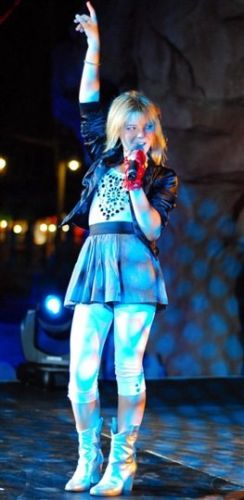The photo captures a young woman in her 20s, performing on stage at night. She stands in dynamic, pop star fashion, holding a wireless microphone in her left hand which is adorned with a red glove. She points her right hand skyward, striking a confident pose. Her blonde hair cascades around her shoulders, complementing her outfit: a black leather jacket pulled up above the elbows, a white shirt adorned with a black design vaguely resembling a triangle with a central circle, a short gray skirt with a black waistband, and off-white leggings ending just below her knees. She completes her look with gold high-heeled booties. She appears to be lit by a projector, casting round and square shapes around her, adding a dramatic flair to her nighttime performance.